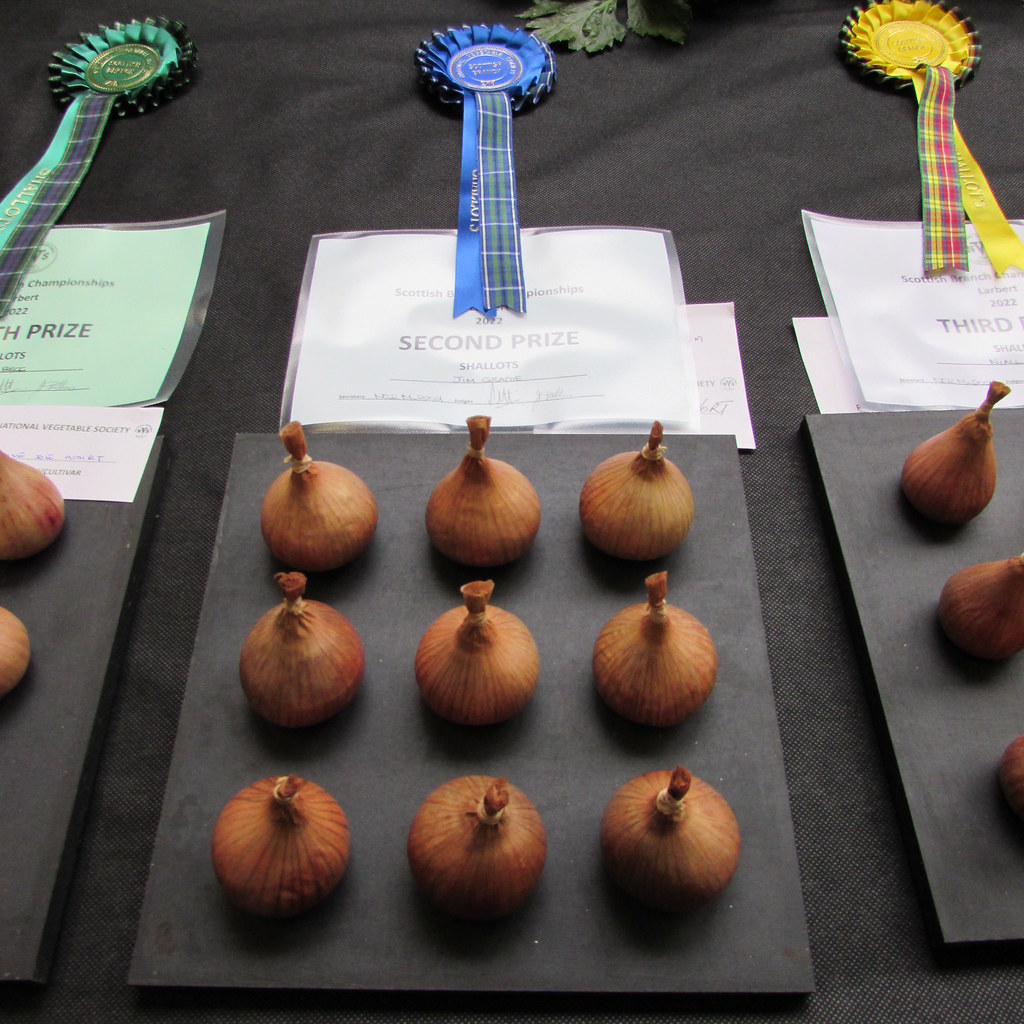The photograph captures a meticulously arranged display of shallots on a table draped with a black tablecloth, suggesting an agricultural contest, possibly a 4-H or farmer's convention. Central to the image is a square black plate showcasing nine plump, brownish-orange shallots, labeled as winning second prize with a blue ribbon and a certificate reading "Shallots." This plate is positioned at the bottom center, with its award indicated at the top center of the photo. Flanking this central plate are two additional plates, each bearing shallots. The plate on the right, marked with a yellow ribbon for third prize, and the plate on the left, adorned with a green ribbon, though the prize ranking remains unclear. The photograph emphasizes the visual appeal and quality of these shallots, celebrating their prize-winning status in the competition.